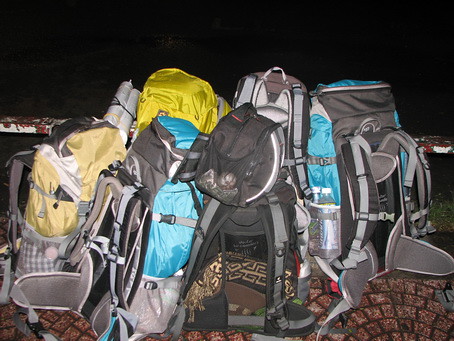The photograph depicts a realistically captured scene set against a jet-black background, indicating it was taken at night. The foreground reveals a plaza or surface covered with reddish and white brick tiles laid out in a circular pattern. Centrally, there is a cluster of six hiking backpacks of varying colors and conditions, predominantly black and gray, but including striking hues of bright yellow, light aqua blue, and a buttery yellow. These backpacks are well-used, featuring multiple straps for shoulders and waists, various buckles, and additional storage pouches. Some have water bottles or beverage containers in their side pockets, and one backpack appears to contain a folded tan and brown blanket. The backpacks, standing upright and leaning against each other, are positioned near a short wall, silhouetted starkly against the dark, featureless backdrop.